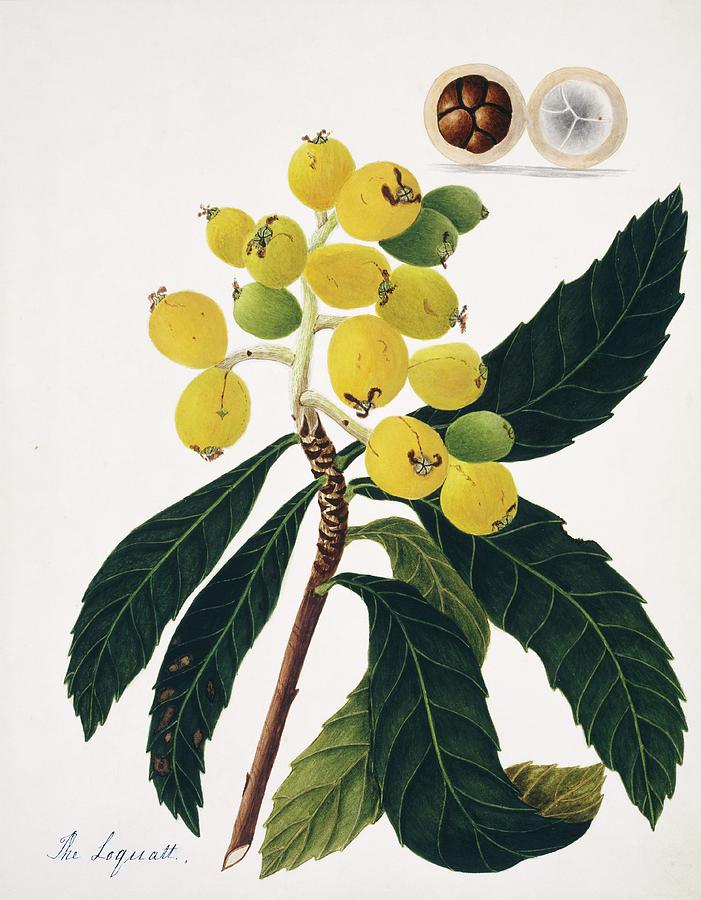This detailed drawing depicts a distinctive plant displayed on a rectangular canvas, with the longer sides twice the length of the shorter sides. The background is a soft tannish-white color, creating a subtle yet effective contrast for the artwork. In the bottom left corner, a cursive signature reads "the loquat," indicating the plant type.

At the base of the illustration, a cut branch reveals its brown exterior and white interior. As the branch ascends, it supports several large, elongated green leaves, richly detailed with light green veins against a dark green backdrop. Near the top, the branch transitions to a white color and bears numerous lemon-shaped fruits, varying in color from yellow to green. 

Notably, around the upper right section of the image, there are two inset circles. One circle appears to show the seed of the loquat fruit, while the other presents a designed accent, suggestive of the fruit's internal structure. These details, combined with the intricate depiction of the leaves and fruits, illustrate the artist's careful attention to botanical accuracy and texture, characterized by the pastel tones and fine line work that suggest colored pencil as the medium. The signature and the finely executed sketch suggest the artist's intent to provide a detailed and lifelike representation of a loquat branch in all its natural intricacy.